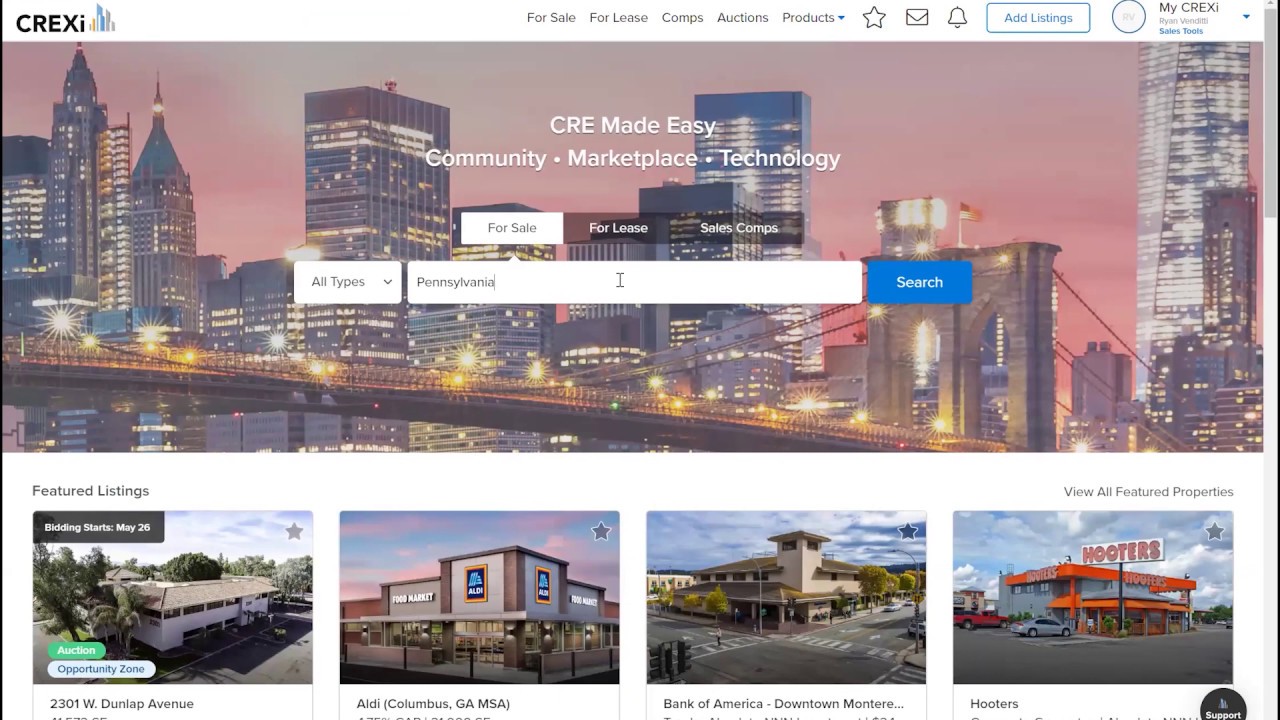This is a detailed screenshot of the CREXI platform interface. The logo, "CREXi," features a capital "C-R-E-X" followed by a lowercase "i," next to a small icon depicting a colorful city skyline, located in the upper left-hand corner. To the right of the logo, there is a horizontal menu with clickable links: "For Sale," "For Lease," "Comps," "Auctions," and "Products." To the far right of these menu options, there is a series of icons and text: a star, an envelope icon representing email, an alert bell, and a white rectangle with blue text that reads "Add Listings." Proceeding further right is a gray circle with the initials "RV," followed by black text reading "My CREXI," underneath which the username "Ryan Venditti" is displayed in small, grayed-out text. Directly below this username, in blue text, it reads "Sales Tools."

The background image beneath this header is a vibrant depiction of a city skyline at either dusk or dawn. The buildings, adorned with numerous lights, stand illuminated against a reddish-tinged sky. Prominently featured within the image is a bridge that partially spans the view, with densely-packed, well-lit buildings forming an evocative urban backdrop.